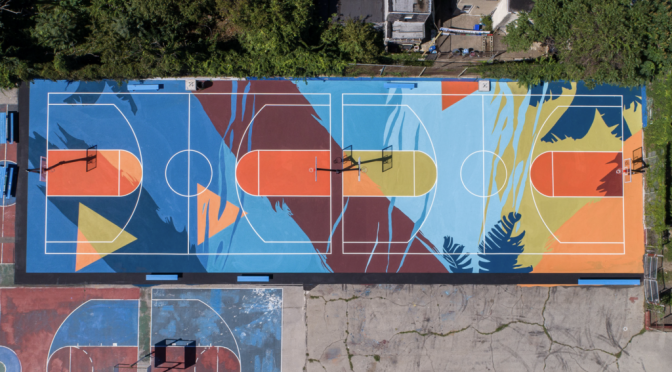This aerial view captures a vibrant, multicolored basketball court nestled within a lush, green landscape. At the center of the image, the basketball court stands out with its striking colors—varying shades of blue, orange, yellow, and sections of green. The court is decorated with darker blue palm tree leaves and features multiple white lines and four basketball hoops, indicating two side-by-side courts.

The courts exhibit a unique, non-regulation pattern, almost resembling a stylized surfboard. The play area beneath the hoops is distinctly orange, and various geometric shapes, including triangles, add to the artistic design. Surrounding the courts is a mix of cracked concrete and residential areas, with a partially visible white house nestled in the greenery above. The image hints at additional courts beyond the visible area, suggesting a larger recreational space. Overall, the scene blends the vibrancy of recreational sport with the tranquility of its surrounding natural and residential environment.